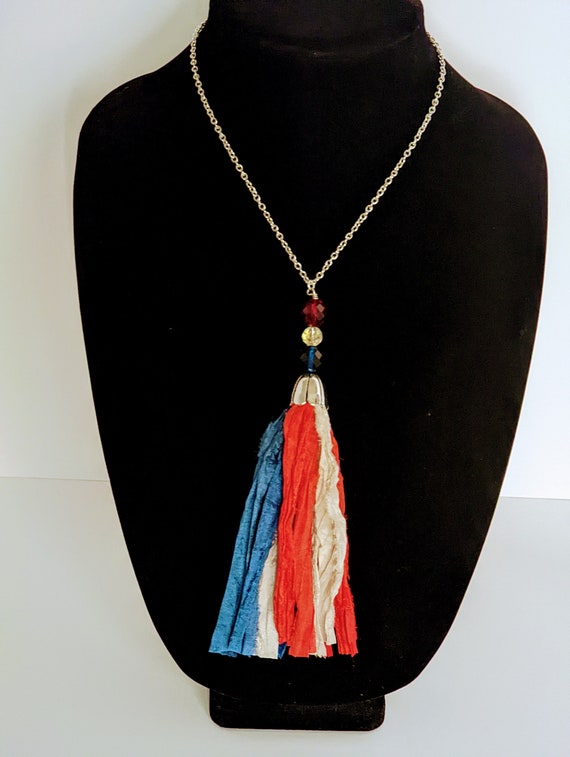Displayed on a black jewelry bust against a white background, the centerpiece is a striking gold necklace featuring a pendant with distinct elements. At the top of the pendant, immediately below the simple gold chain, lies a dark red gem, followed by a yellow gem, and then a dark blue gem arranged vertically. Beneath these gems hangs a colorful tassel, secured by a gold piece of metal. The tassel itself is composed of intertwined fabric in varying hues—red, cream, and blue—resembling wrinkled, fan-like layers or folded rags. These colors echo the gems above, creating a cohesive, vibrant visual appeal. The bust, serving as the display medium, focuses attention on the intricate details of the necklace, from the shimmering chain to the multicolored fabric tassel.